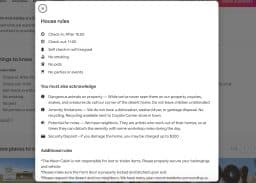The image depicts a white-background pop-up overlay that is partially obscuring the underlying content, turning the background a gray color. Despite the image being blurry, some elements are discernible. In the upper left corner of the pop-up, there is a small circle surrounded by white space and outlined with a gray border. Below this border, a black line appears faintly, potentially signaling an area for entering first and last names.

Further down, there are visible sections with text: one section has regular text, another features bold words followed by bullet points, suggesting a list format, and a third section also contains bold text. Although the titles and contents of these sections are unreadable due to the blurriness, it is clear that the pop-up has three distinct parts.

In the background, on the right-hand side, the top part of the overlay's border is tinged with a magenta paint-like color, contrasting with the white space above it. Overall, the image combines a mixture of gray, white, and magenta hues, and the content appears to be a form or interactive element, though the specifics are unclear due to the lack of clarity in the image.